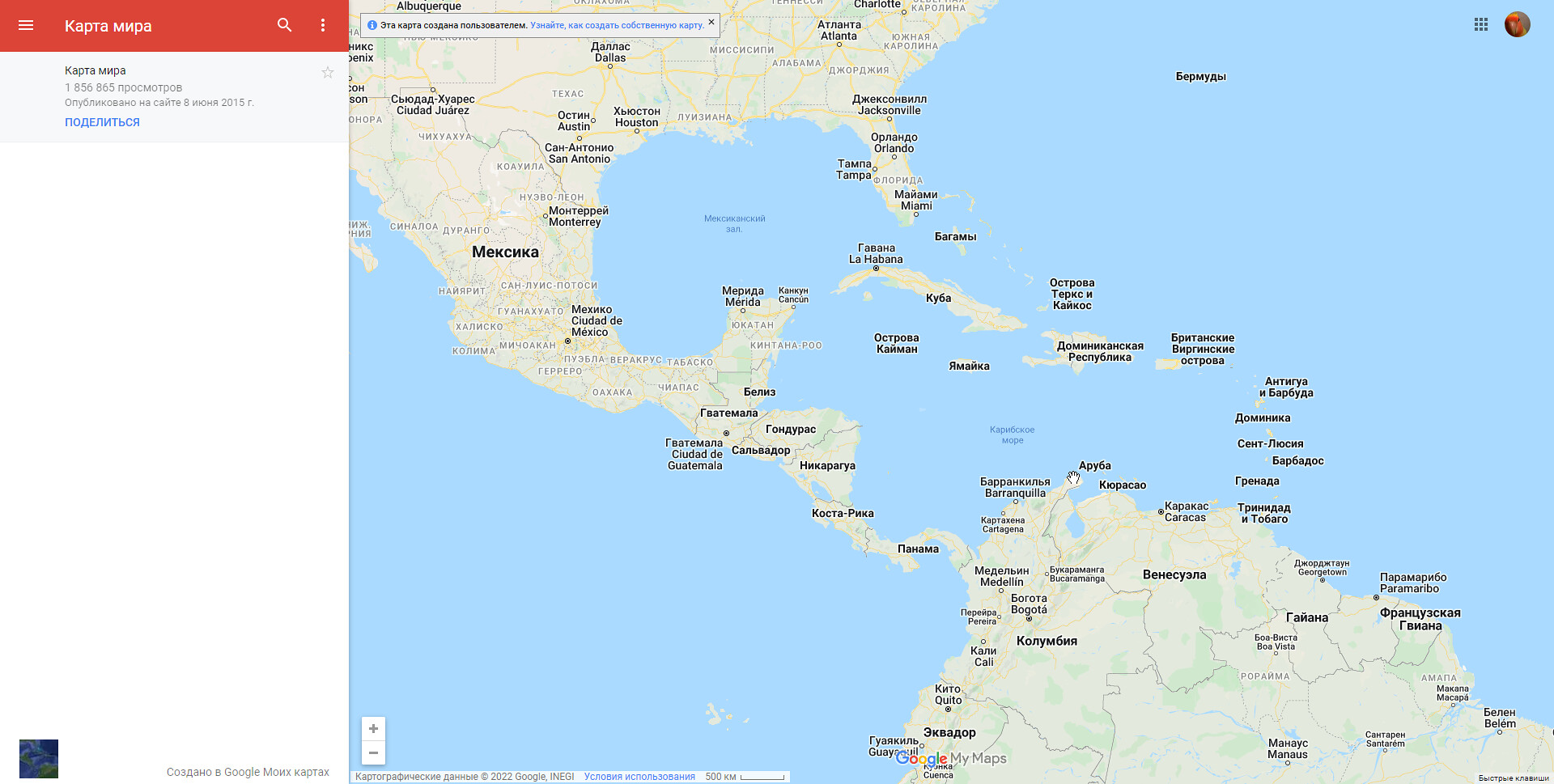The image showcases a detailed map of the Southern United States and the northern part of South America, with the intervening ocean. The map is primarily labeled in a foreign language, whose identity is unknown to the viewer, although it includes some English annotations for specific cities. 

The landmasses are depicted in a light grayish color. Starting from the top, notable English-labeled cities in the Southern United States include Albuquerque, Charlotte, Dallas, Austin, Houston, Jacksonville, Orlando, Tampa, Miami, and Monterrey. Moving down into Central America, the map identifies countries and regions with names in the foreign language, making them unrecognizable except for Guatemala, which is spelled out in English.

The oceans are colored a light blue and seem labeled in the foreign language as well. Various islands are also named in this other language. Nevertheless, once reaching South America, certain English city labels become noticeable again, such as Georgetown and Manaus. There is a peculiar red label on the left side of the map that reads "КАРТА МИРА," written in the foreign script.

At the bottom of the image, there is a label indicating the source as "Google My Maps," suggesting the map was generated or customized using Google Maps software.